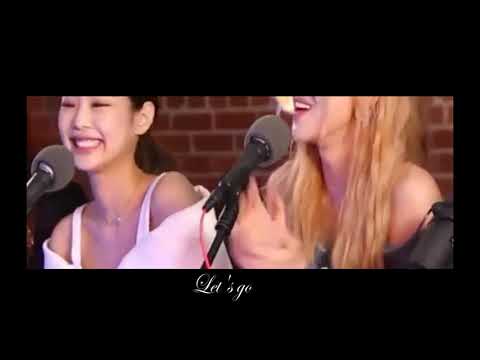The image features a rectangular background with prominent black borders: thick black sections at the top and bottom, and thinner black lines along the left and right edges. The main picture showcases two women with a red brick wall behind them, giving it a lively, urban atmosphere. On the left, there is an Asian woman, possibly Korean, with dark hair, wearing a white tank top paired with a shawl. She has a necklace on and is smiling as she sings into a microphone. Her image is displayed from her forehead to her chest, partially cut off, emphasizing her singing posture and expression. To her right, another woman with long blonde hair, also smiling, wears what appears to be a sleeveless dress outfit with a blue hue. She holds a microphone with a pink cord and her image is shown from her lips down to her chest, as if she is singing or clapping. Both women seem to be members of a music group, potentially a K-pop band, given their styled appearance and expressive demeanors. At the bottom of the image, there is cursive white text that reads, "Let's Go," suggesting an enthusiastic or motivational theme.